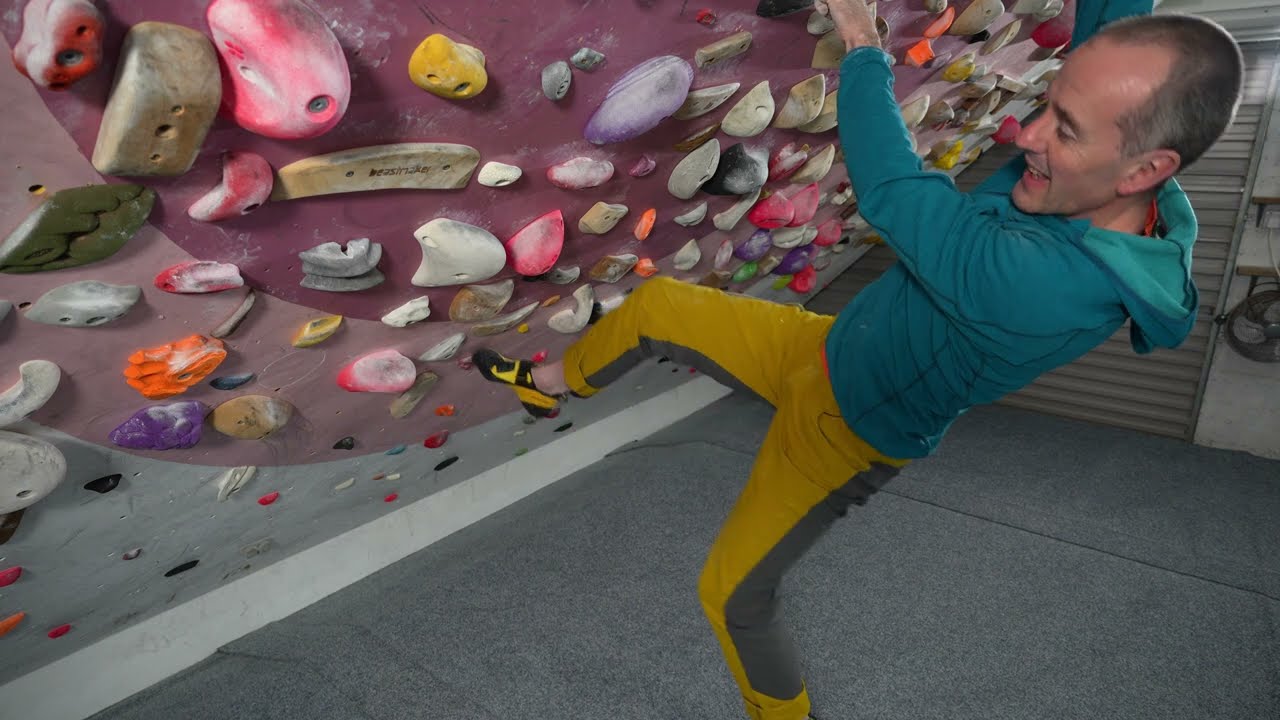This photograph captures a balding man in his late 40s enthusiastically engaged in indoor rock climbing. He is clad in a teal hoodie and distinctive yellow and gray slacks, specially designed for climbing, along with the appropriate rock climbing shoes. The indoor climbing wall he's tackling is fitted with a myriad of vividly colored rock grips—pink, yellow, purple, white, green, and more—providing both aesthetic appeal and varied gripping options. Positioned on the wall, the man has both hands gripping the colorful holds, with his right foot securely placed on another. His left foot remains on the low-pile gray carpeted floor, indicating he's just about to propel himself upward. The angled, almost fisheye perspective of the camera accentuates his enthusiastic smile as he contemplates his ascent. Additionally, the background reveals a metal door and a fan bolted to the wall, enhancing the sense of an indoor climbing gym environment.